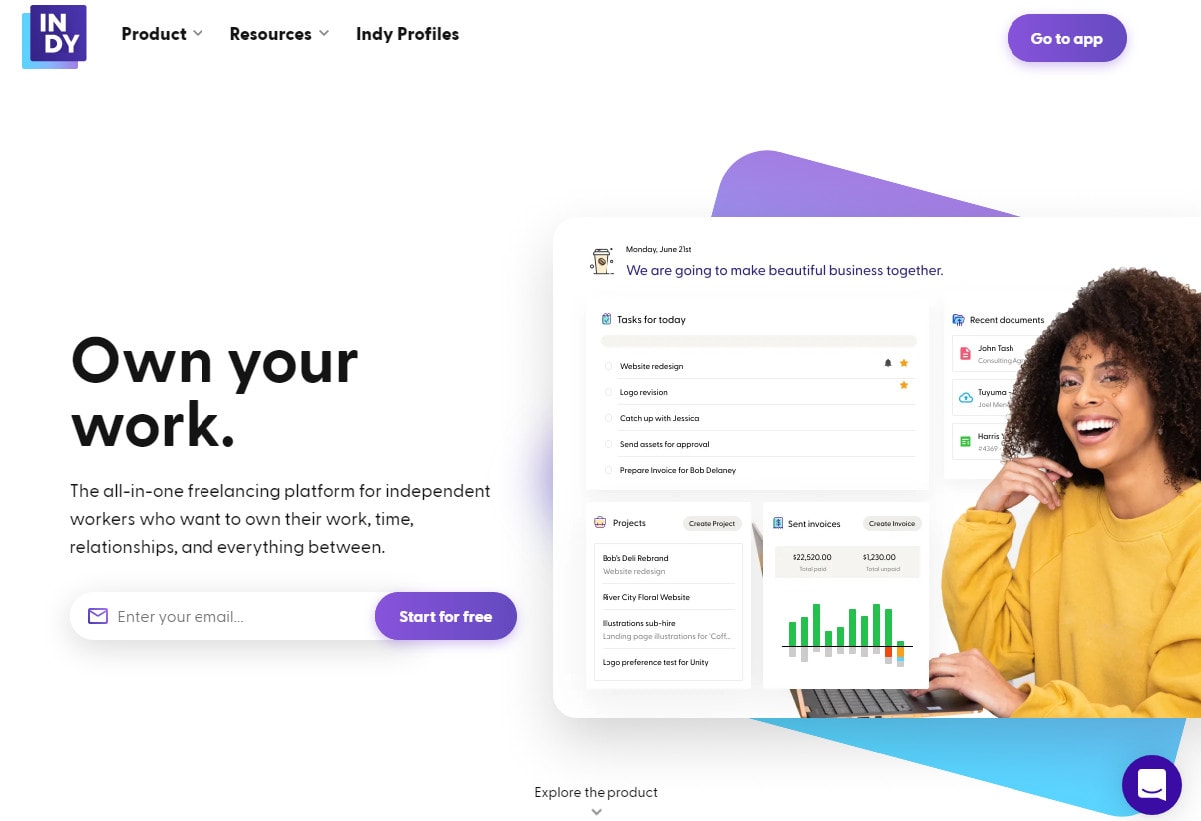This is a detailed description of a screenshot depicting the Indie web page:

At the top left corner of the page, the Indie logo is prominently displayed. This logo features a unique design comprising a light blue box and an offset purple box with the word "INDY" centered within the boxes. Adjacent to the logo, there are navigation options labeled "Products," "Resources," and "Indie Profiles."

On the right side of the header, there is a circular button inscribed with the text "Go to App," providing a clear call-to-action for users to access the application. The entire page is set against a clean white background.

Centrally located and aligned to the left, a bold headline reads "Own Your Work" in large black letters, capturing the primary message of the platform. Directly below this, a subheading describes Indie as "the all-in-one freelancing platform for independent workers who want to own their work, time, relationships, and everything in between."

Further down, there is an input field inviting users to "Enter your email and start for free," encouraging instant engagement.

To the right of these textual elements, there is a white square image featuring a woman typing on a computer, with the visual effect of the woman appearing to emerge from the white box. Along the left side of this image, a motivational statement reads, "We are going to make a beautiful business together." Additionally, overlaid on the image are various graphical elements and sections labeled "Tools for Today," "Projects," and "Documents," hinting at the features offered by the platform.

Lastly, at the bottom right corner of the page, a small purple bubble with a chat box icon and a smiley face indicates the presence of a live support chat feature, ready to assist users with any inquiries they may have.